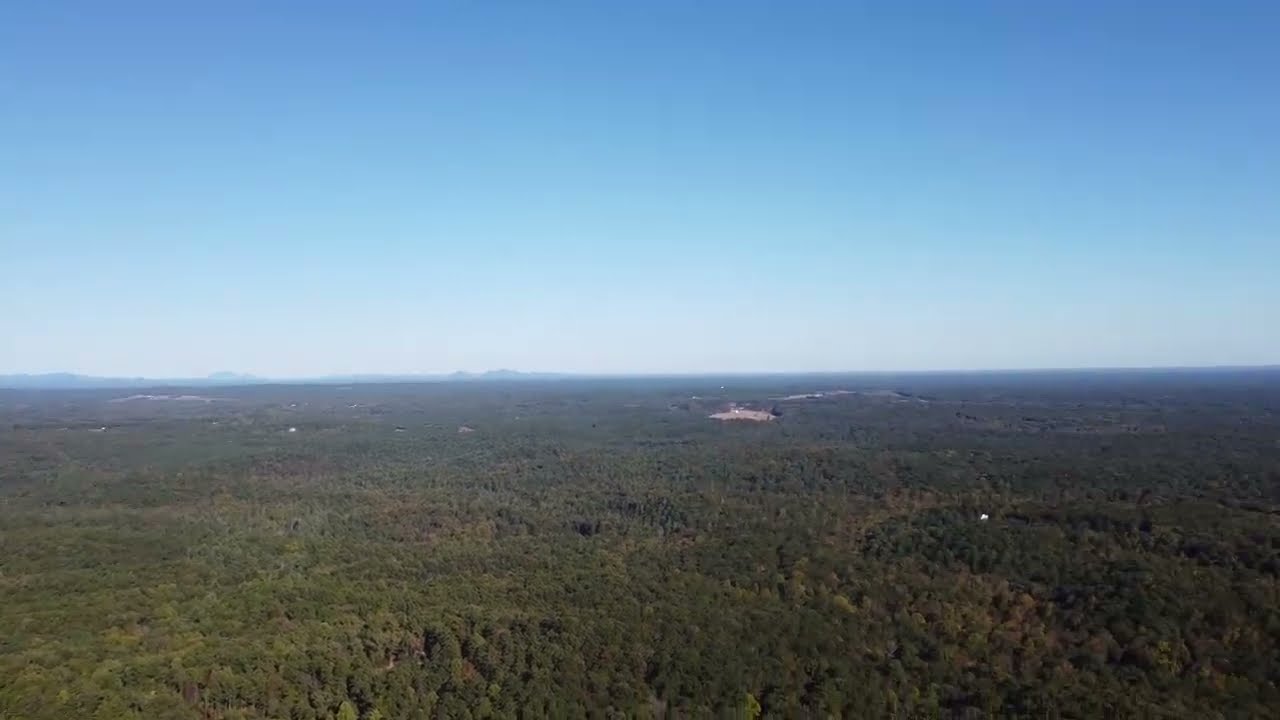The image presents an expansive aerial view of a dense forest with various shades of green dominating the bottom half of the frame. The forest appears vast and unbroken, densely packed with pine and other trees, creating a thick canopy of foliage. In the middle of the image, there's a brown open patch that may indicate a clearing or a sandy, dirt area. Towards the left midsection of the image, the silhouette of distant mountains or hills is faintly visible on the horizon, shrouded in a hazy atmosphere that suggests their considerable distance. The top half of the image is filled with a vivid, deep blue sky, devoid of clouds, contributing to the clarity and brightness of the scene. The overall setting portrays a serene and untouched natural landscape with no signs of human presence, roads, or structures, emphasizing its tranquility and remoteness.